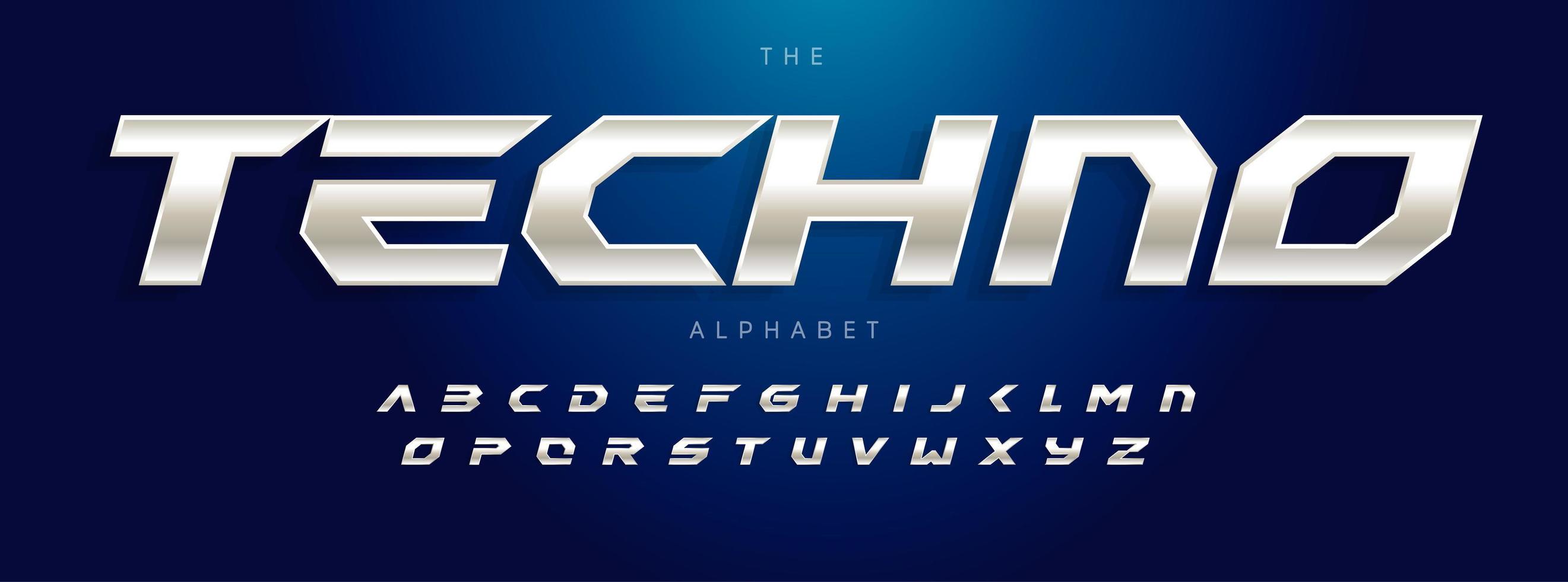The image appears to be an advertisement featuring the words "The Techno Alphabet" in vivid, eye-catching fonts against a gradient blue background that transitions from dark blue on the sides to a lighter shade in the middle. The title "THE TECHNO" is prominently displayed in large, shiny, silver lettering, styled in a blocky, cyberpunk-inspired font. The letters are characterized by their angular, geometric shapes, where for instance, the 'O' resembles a hexagon and the 'A' looks like an inverted 'V'. Below "TECHNO," the word "ALPHABET" appears in a similar but smaller light blue capital font. Beneath the title, the entire alphabet from A to Z is showcased in the same techno font, with each letter capitalized and designed uniquely to maintain the font’s futuristic and mechanical aesthetic. The detail-oriented design has the letter 'B' crafted to resemble a '3', and the letters 'HIJK' arranged to appear like a less than sign, demonstrating the unique and consistent style of the typeface. Overall, the image strikingly combines text and design elements to create a visually compelling example of a high-tech, modern alphabet.